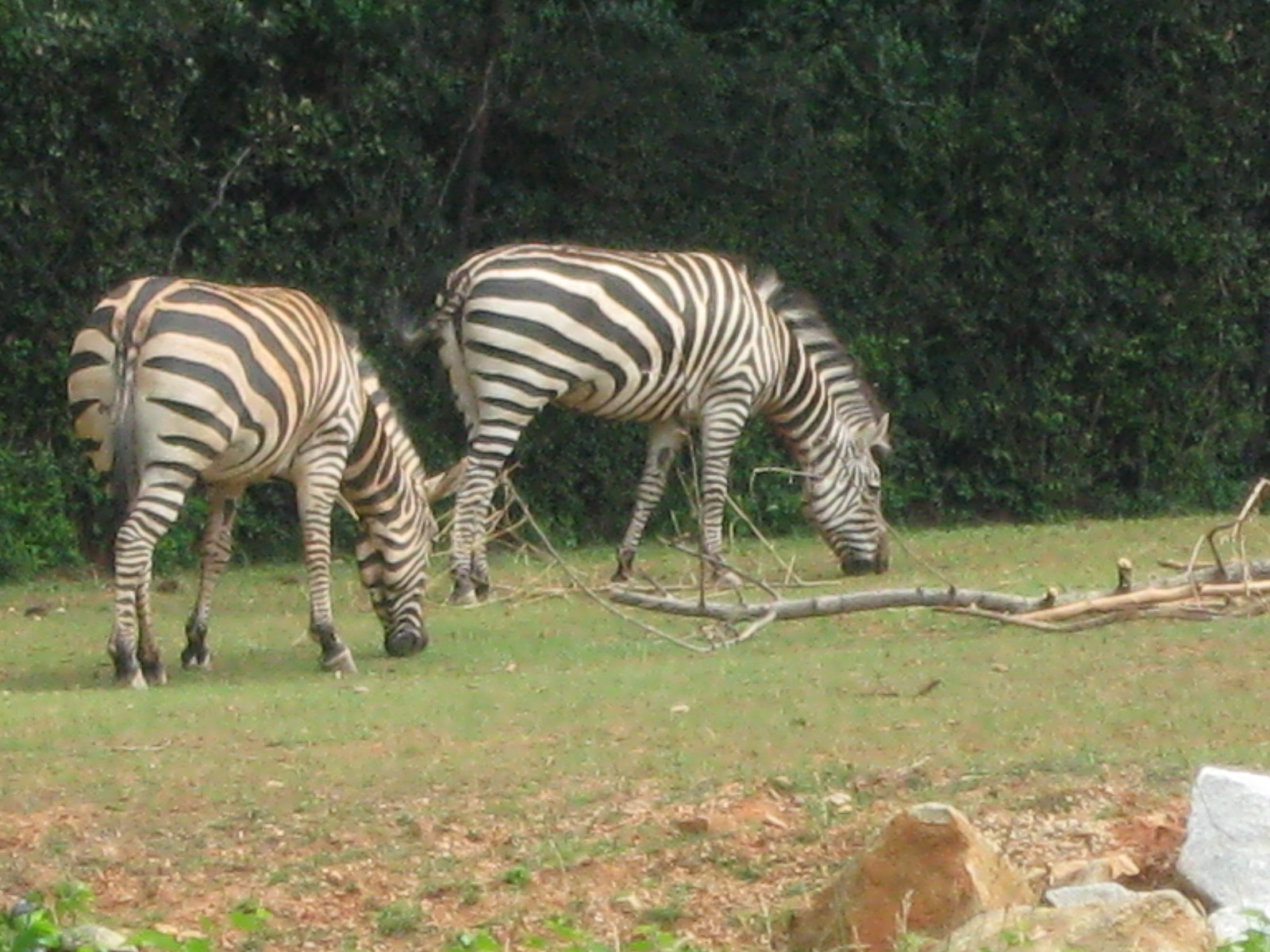A vivid color photograph showcases two zebras standing on a grassy patch, both facing to the right with their heads and necks bent down as they graze. The lush green grass dominates the scene, but there are also notable patches of brown earth and reddish clay. A large, gray, horizontal tree branch lies across the center of the picture, to the left of the zebras. The background is entirely obscured by a dense wall of dark green trees or shrubbery, creating a natural barrier. In the lower right corner, a collection of large rocks in varying shades—rust brown, tan, beige, and almost white—add texture to the scene. Some hints of exposed reddish earth suggest the zebras might have recently taken a dust bath. Overall, the zebras appear to be in a controlled environment, possibly a zoological park.